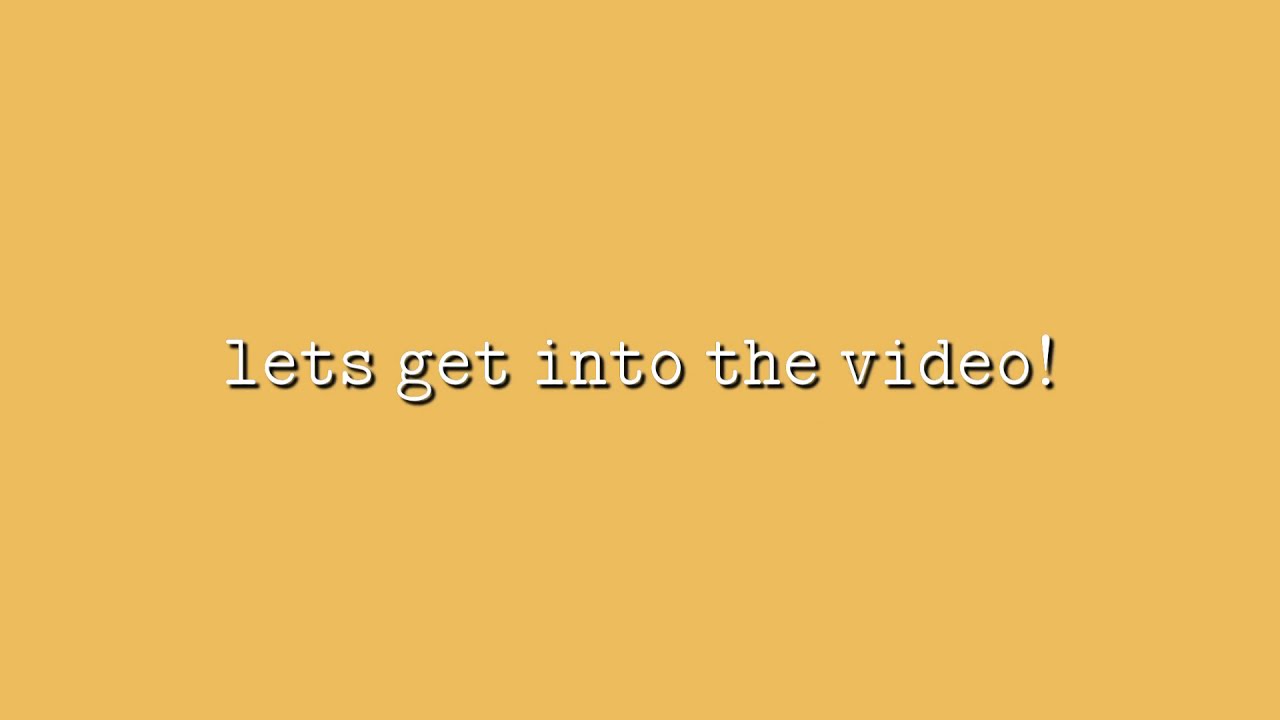The image features a horizontally oriented rectangle, approximately twice as wide as it is tall, with a solid light brownish-yellow background, reminiscent of butter but slightly darker. In the center of the image, in a single line of lowercase white letters shadowed in black for a subtle 3D effect, there's the phrase "let's get into the video!" The text is clear and unadorned, without any apostrophe in "let's." This type of image could serve as an introductory frame in a YouTube video, marking the transition from the opening segment or ads to the main content. The simple yet visually distinct design ensures that the message stands out against the warm background, guiding viewers seamlessly to the core of the video.